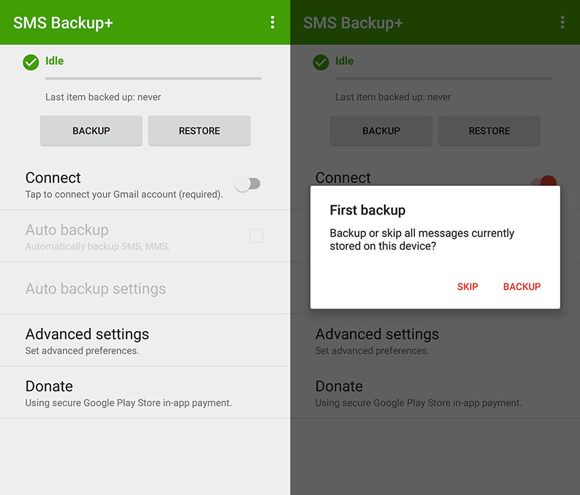This image is a split-screen screenshot of an SMS backup application, showcasing two different states of the app interface. Both sides share similar elements but with distinguishable differences, particularly an error message and a dulled appearance on the right side.

At the very top of both sides, there is a green header with the text "SMS Backup Plus" displayed in white, accompanied by a vertical trio of dots on the right. Directly below, a green checkmark is followed by the statuses "Idle" and "Last item backed up: never" written in dull white text.

The interface includes two prominent gray rectangles labeled "Backup" on the left and "Restore" on the right. Below these buttons, it instructs users to "Connect," requiring a tap to link with a Gmail account. Adjacent to this is a white circular slider control that can be toggled to the right to turn on.

Midway down, in very light gray text, it reads "Auto backup: automatically backup SMS, MMS." Below this is a black text header for "Auto backup settings," followed by "Advanced settings: set advanced preferences and donate using secure Google Play in-app payment."

The right side of the image is further distinguished by a white rectangle with the header "First backup." This section gives users the option to "Backup or skip all messages currently stored on device," with two red buttons at the bottom right: one labeled "Backup" and the other "Skip."

The entire right half of the image is covered with a dark gray overlay that mutes the colors, making it harder to discern details and providing a visual indication of an error or inactive state.